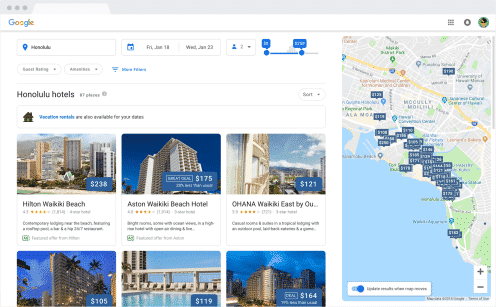This image captures a screenshot of a web browser displaying the Google search results page for hotel bookings in Honolulu, Hawaii. A user is searching for accommodation from Friday, January 18th to Wednesday, January 22nd, for two people with a specified budget. Evidently, there are 97 or 87 hotel options available, though the exact number is written in a small font that is difficult to read.

Prominently featured at the top of the results is the Hilton Waikiki Beach Hotel, priced at $238 per night. Accompanying the price is a small image of the hotel, a brief description consisting of two lines, and its star rating. 

Directly below this, the Aston Waikiki Beach Hotel is highlighted, marked down by approximately 20% and available at $175 per night. This listing also includes a photograph and a short description.

The third option shown is the Ohana Waikiki East by Kew Hotel, also accompanied by an image and a brief overview.

At the bottom of the screenshot, additional hotel options are partially visible, although the full details are cut off.

On the right side of the page, there is an interactive map displaying the geographic locations of all the hotels listed, with their nightly rates clearly indicated. This map provides a visual aid to help users understand where the hotels are situated within Honolulu.